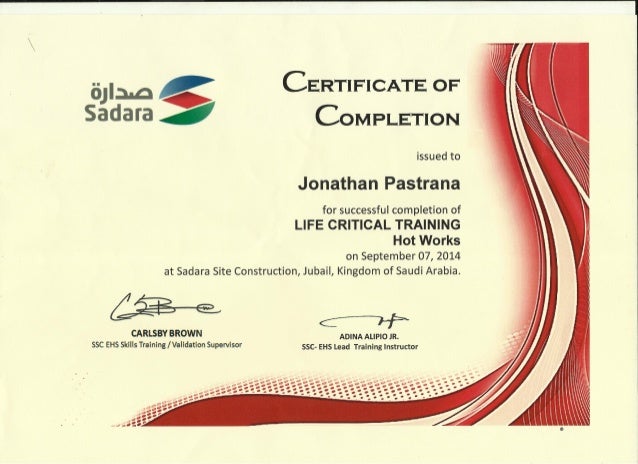This image captures a detailed Certificate of Completion issued to Jonathan Pastrana for the successful completion of Life Critical Training in Hot Works on September 7, 2014, at the Sadara Site Construction in Jubail, Kingdom of Saudi Arabia. The certificate is printed on light beige paper with a sophisticated artistic design, featuring red and various shades of red swirling patterns forming a vertical border along the right side, extending into a backwards L shape at the bottom. The document includes a corporate logo positioned at the top-left corner, which is a combination of blue, red, and green shapes with the word "Sadara" beside it and some non-English text above. This comprehensive certificate lists the names of key personnel: Carlsby Brown, SSC EHS Skills Training Validation Supervisor, and Adina Alipo Jr., SSC EHS Lead Training Instructor, both of whom have signed it at the bottom. Measuring approximately five inches by five inches, the document's detailed layout and corporate elements suggest it may be a carbon copy scan.